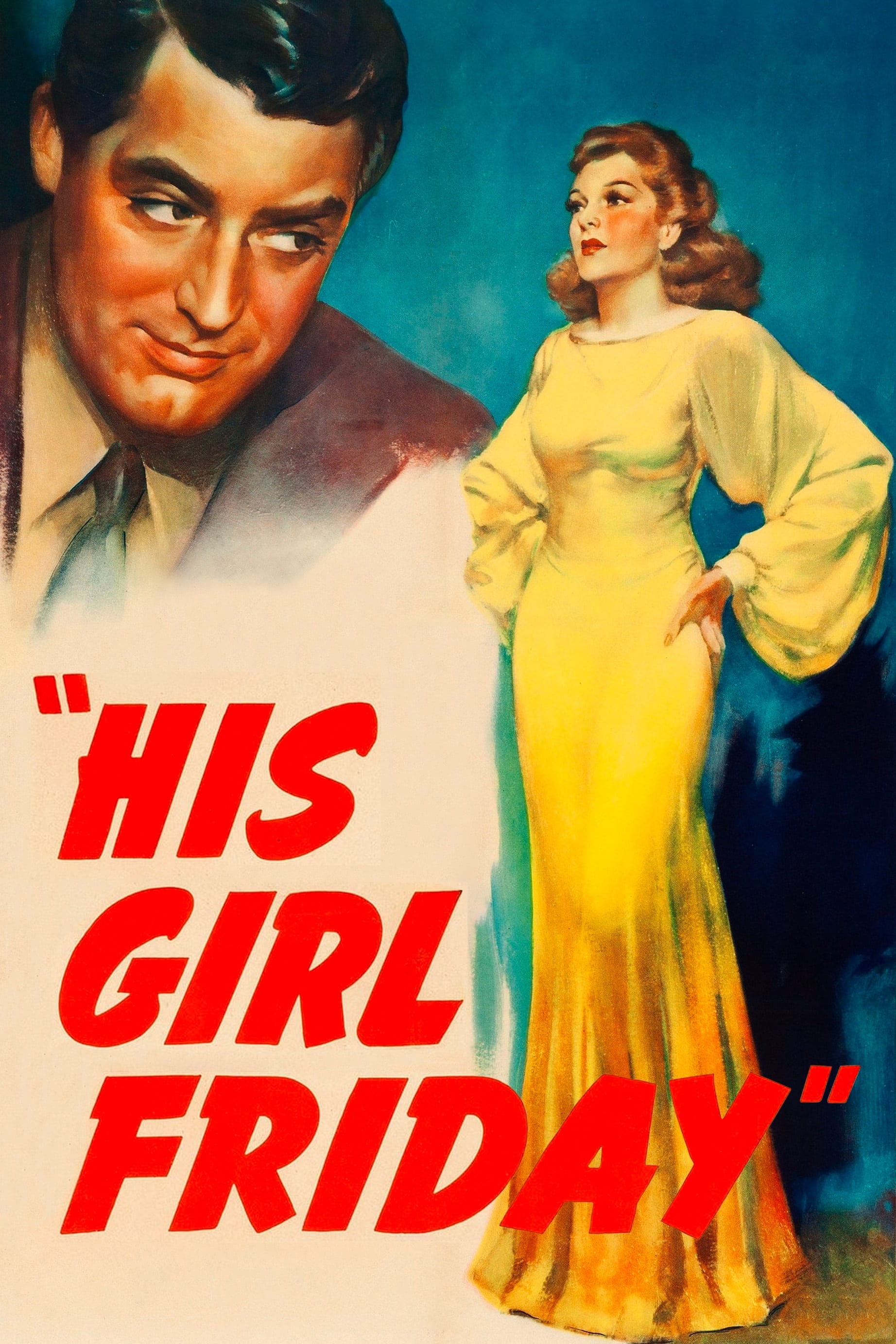The movie poster for "His Girl Friday" prominently features Cary Grant and Rosalind Russell set against a bluish-green background. In the upper left-hand corner, Cary Grant, depicted in a brown suit with a blue or green tie, looks longingly at Rosalind Russell. He has dark hair and appears larger than the woman, with his head and shoulders dominating that section. Rosalind Russell stands in the right-center of the poster, wearing a striking yellow gown that extends to the floor. The dress detail includes puffy sleeves that fitted at the bodice and waist before flaring out at the thighs, transitioning to a darker yellow at the hem. Russell’s red, curly hair complements her confident pose with hands on her hips, casting a shadow on a wall behind her. She seems to regard Grant with a neutral expression. The title, "His Girl Friday," is displayed in bold, bright red letters across Cary Grant's suit, which fades to white to enhance the visibility of the text. This classic design lends a vintage feel, reminiscent of the 1930s or 1940s era, and is clearly meant to draw attention as a movie poster.